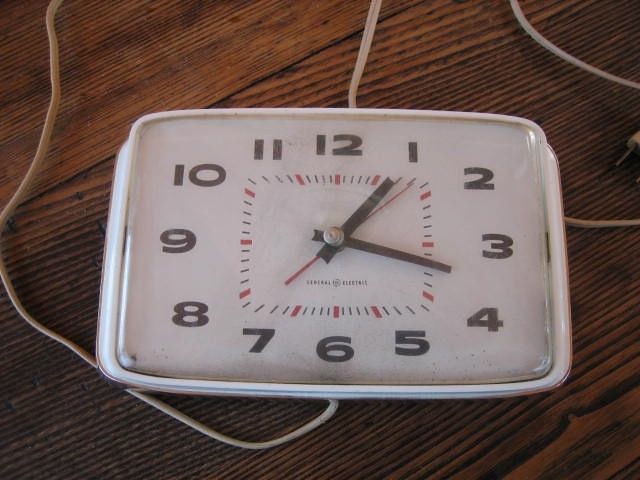This photograph features a vintage, 1970s-era analog alarm clock, positioned on a varnished dark wooden table, which may double as a bedside table. The clock, composed primarily of white plastic, has a somewhat rectangular shape and is enclosed with a clear plastic cover over the face. The clock is powered by a white electric cord with a two-prong plug. The clock face displays black numerals ranging from 1 to 12, accompanied by red lines marking the hours and smaller red dashes for the minutes. The clock’s hands include a large and small hand, both in dark brown or black, and a thin red second hand, all secured by a central silver pin. The current time shows as approximately 1:17, with the second hand positioned around the seven-second mark.